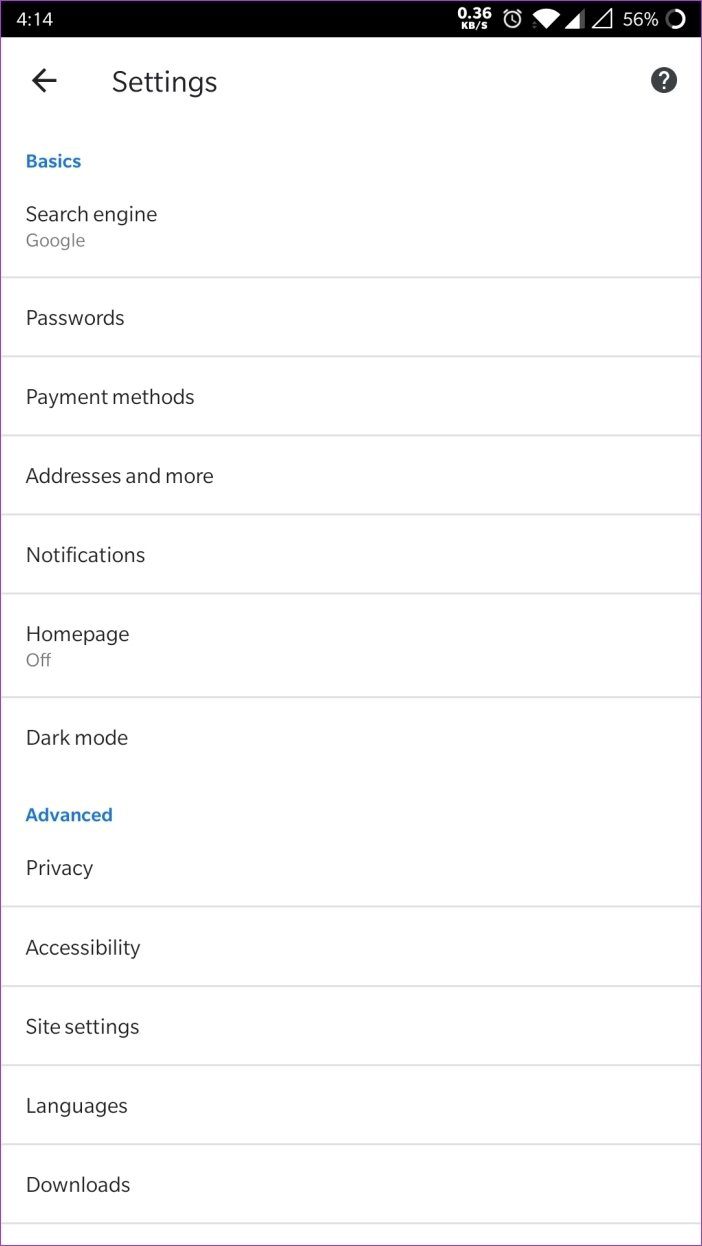The image is a screen capture from a digital device, displaying a settings menu on a white background. At the upper left corner, the word "SETTINGS" is prominently featured in large black text. Below this, a section header titled "BASICS" is written in blue text. Underneath the "BASICS" header, several options are listed in black text, including "SEARCH ENGINE GOOGLE," "PASSWORDS," "METHODS," "ADDRESSES and more," "NOTIFICATIONS," "HOME PAGE," "OFF," and "DARK MODE." Further down, another section header "ADVANCED" is written in blue text. Under the "ADVANCED" section, the options listed in black text are "PRIVACY," "ACCESSIBILITY," "SITE SETTINGS," "LANGUAGES," and "DOWNLOADS."